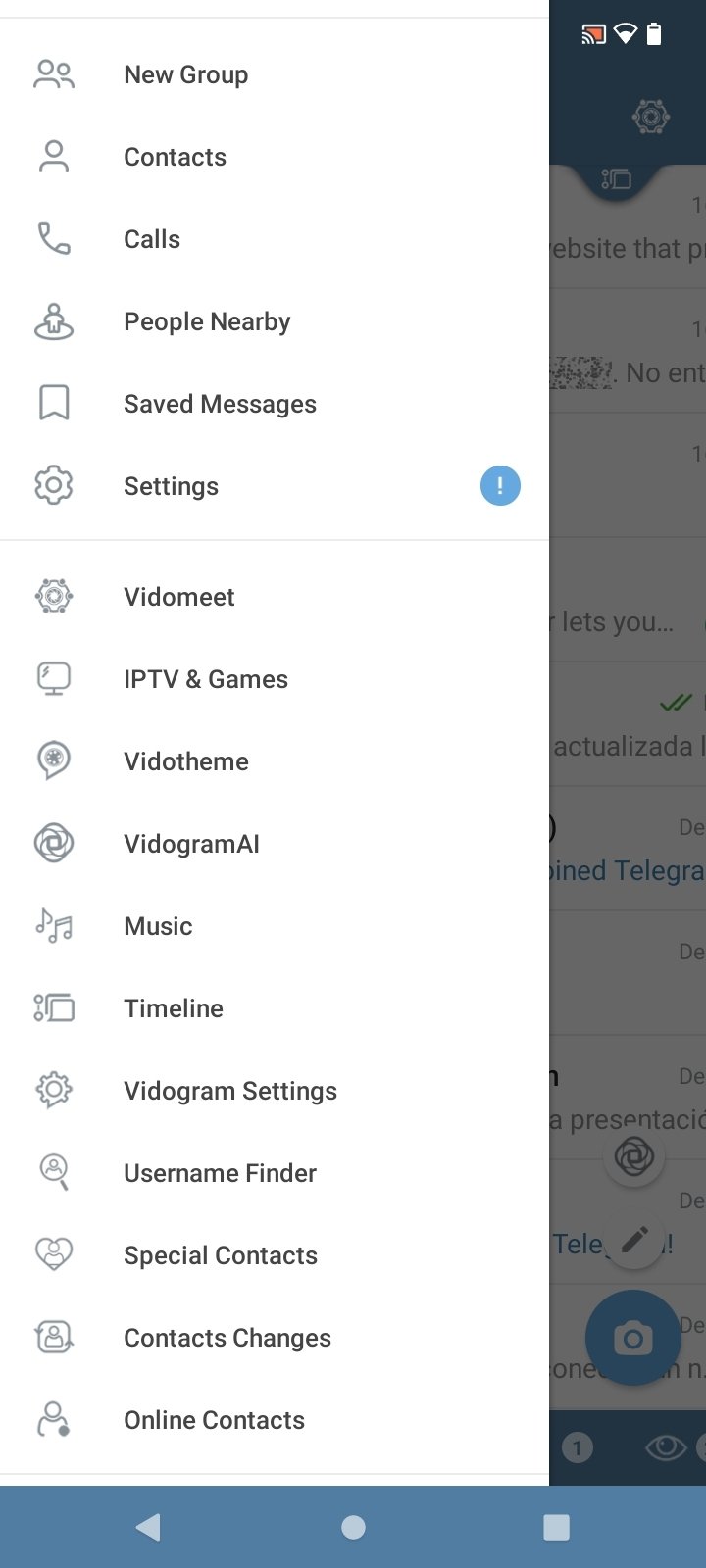The image depicts a smartphone device with a prominently white screen that displays a list of various attributes aligned vertically on the left-hand side. Accompanied by plain black and white icons, the list starts with "New Group," followed sequentially by "Contacts," "Calls," "People Nearby," "Saved Messages," and "Settings." A fine gray line separates these from additional items below, which include "Fiddle Meet," "IPT and Games," "Fiddle Theme," "Fiddlegram AI," "Music," "Timeline," "Fiddlegram Settings," "Username Finder," "Special Contacts," "Contacts Changes," and "Online Contacts."

On the right-hand side of the screen, there is a slightly darkened panel running the full length of the phone, approximately one and a half centimeters wide. At the top of this panel, a Wi-Fi signal indicator and a battery status icon are visible. This panel is somewhat translucent, allowing a glimpse of text underneath, though it is largely obscured by the darker shade. At the very bottom of the screen, a fine blue panel features what appears to be pause and play buttons.